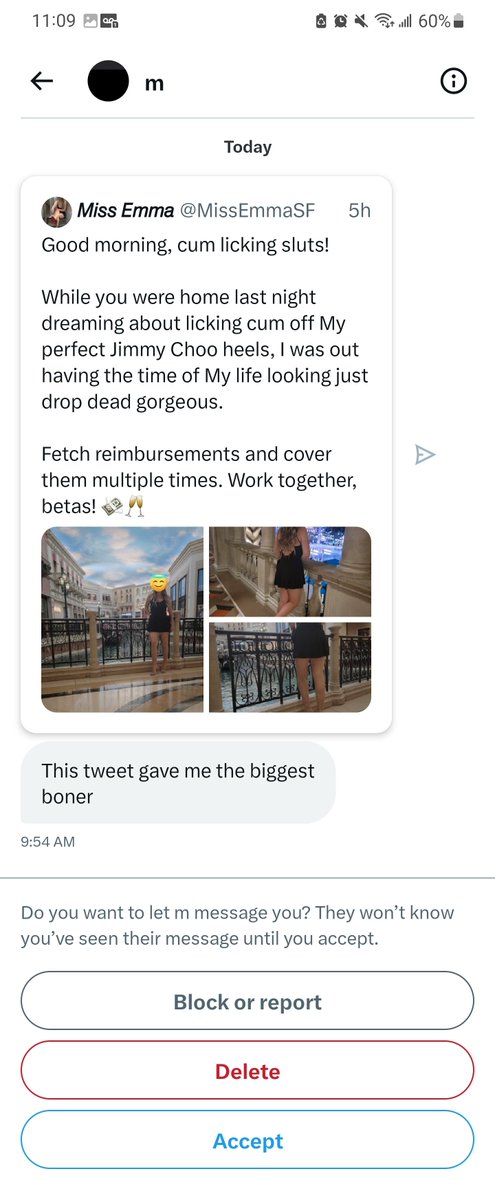Here is a cleaned-up and detailed caption for the described image:

---

A screenshot from a smartphone, featuring a white background with various interface elements. At the top left, the time is displayed as 11:09 AM. To the right of the time, there is a battery icon indicating a 60% charge. Below the status bar, an arrow pointing left is seen next to a black circle with the letter "M" beside it. A light gray separator line follows below.

Underneath the separator, the interface features the word "Today," signaling the current date. Further down, a social media post by a user named Ms. Emma (@MsEmmaSF) is visible, posted five hours ago.

The post begins with "Good morning," followed by an explicit and rude paragraph. Below the text, there are three pictures, one of which is a picture of a girl wearing a short dress. Accompanying the images, the caption under the post reads, "This tweet gave me the biggest V-O-N-E-R."

At the bottom of the post, a notification inquires, "Do you want me to let M message you? They won't know you've seen their message until you accept." Below this query are options to "Block," "Report," "Delete," or "Accept" the message.